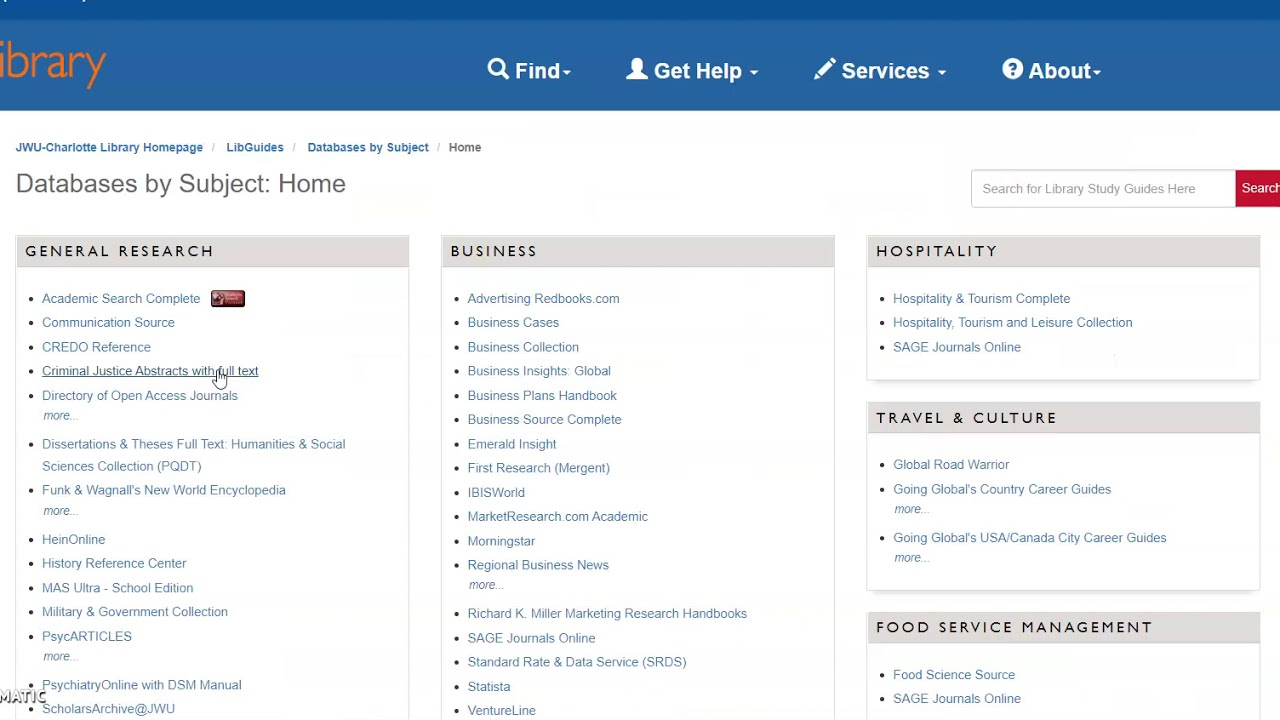The image displays a webpage with a blue banner at the top. On the left side of the banner, the word "Library" is partially visible in red, showing only "B-R-A-R-Y." The banner also features white text with drop-down menus labeled "Find," "Get Help," "Services," and "About." Below the banner, the page has a white background, occupying the main content area.

At the top of this section, there are navigation tools with links titled "JWU.Charlotte Library homepage," "Lib Guidelines," "Database by Subject," and "Home." On the right side, there's a search bar with placeholder text "Search for library study guides here" and a red "Search" button.

Further down the page, on the left, there's a section titled "Databases by Subject, Home," followed by five categories, each headed with a gray bar. The categories are "General Research," "Business," "Hospitality," "Travel Culture," and "Food Service Management." Under the "General Research" category, with a teal-colored background and bullet points, the listed resources include "Academic Research Complete," "Communication Source," "CREDO Reference," "Criminal Justice Abstracts with Full Text," where the cursor appears as a hand, indicating a click on the underlined link, "Directory of Open Access Journals," "More," "Destinations and Themes," "Full Text," "Humanities and Social Studies," "Science Collections," and "PQDT."